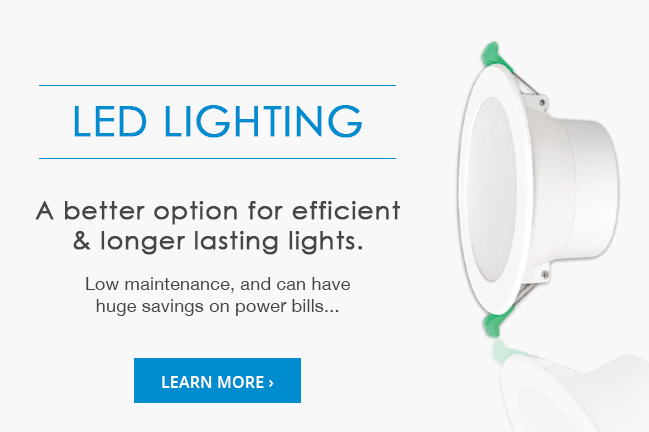The image showcases a promotional banner for LED lighting, commonly seen on computer or tablet screens. The banner features a horizontal gray box with text and a graphic.

In the top-right corner, a bold blue line of text reads "LED LIGHTING" in all caps. Below that, a secondary line in black mixed-case lettering states, "A better option for efficient and longer-lasting lights." Followed by another line emphasizing "Low maintenance and can have huge savings on power bills."

At the bottom of the text section, there is a clickable "Learn More" button, accompanied by an arrow, inviting the viewer to explore additional information about the LED lighting.

To the right of the textual information, the graphic depicts the LED light itself. The depicted LED light has an oval shape with a canister-like back. The installation mechanism includes two green attachments, positioned at the top and bottom of the light, presumably for securing the light into a ceiling. The LED light also casts a reflection on a mirrored or reflective surface, enhancing its visual appeal.

Overall, the advertisement highlights the benefits of LED lighting, focusing on efficiency, longevity, low maintenance, and significant power bill savings.